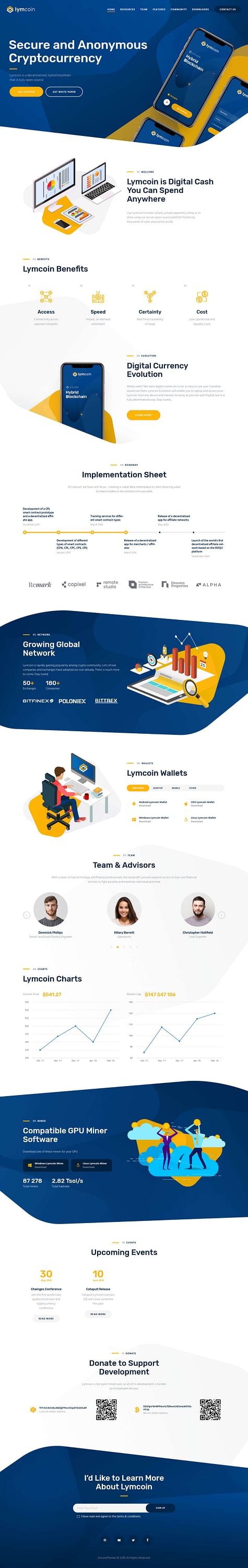The web page, which appears to be associated with a potential builder's merchant, features a complex layout with multiple sections. The top of the page includes four long, irregularly shaped slots spanning horizontally across it, making navigation challenging. Below the first slot, there are smaller images accompanied by text, providing additional information or context.

Further down, a smaller blue slot with text appears, leading into another large section that possibly showcases buildings or architectural structures. This large section could serve as a visual highlight or feature area.

Within the content, there are also thumbnail images of three individuals: a man, a woman in the center, and another man. Additionally, the page includes an intriguing image of a couple standing, seemingly, in a pool of blue water bordered with yellow hues. Despite the aquatic setting, their attire suggests they are not dressed for the beach, adding an element of mystery to the image.

The overall layout and design are intricate, potentially overwhelming and difficult to interpret without prior knowledge or context.